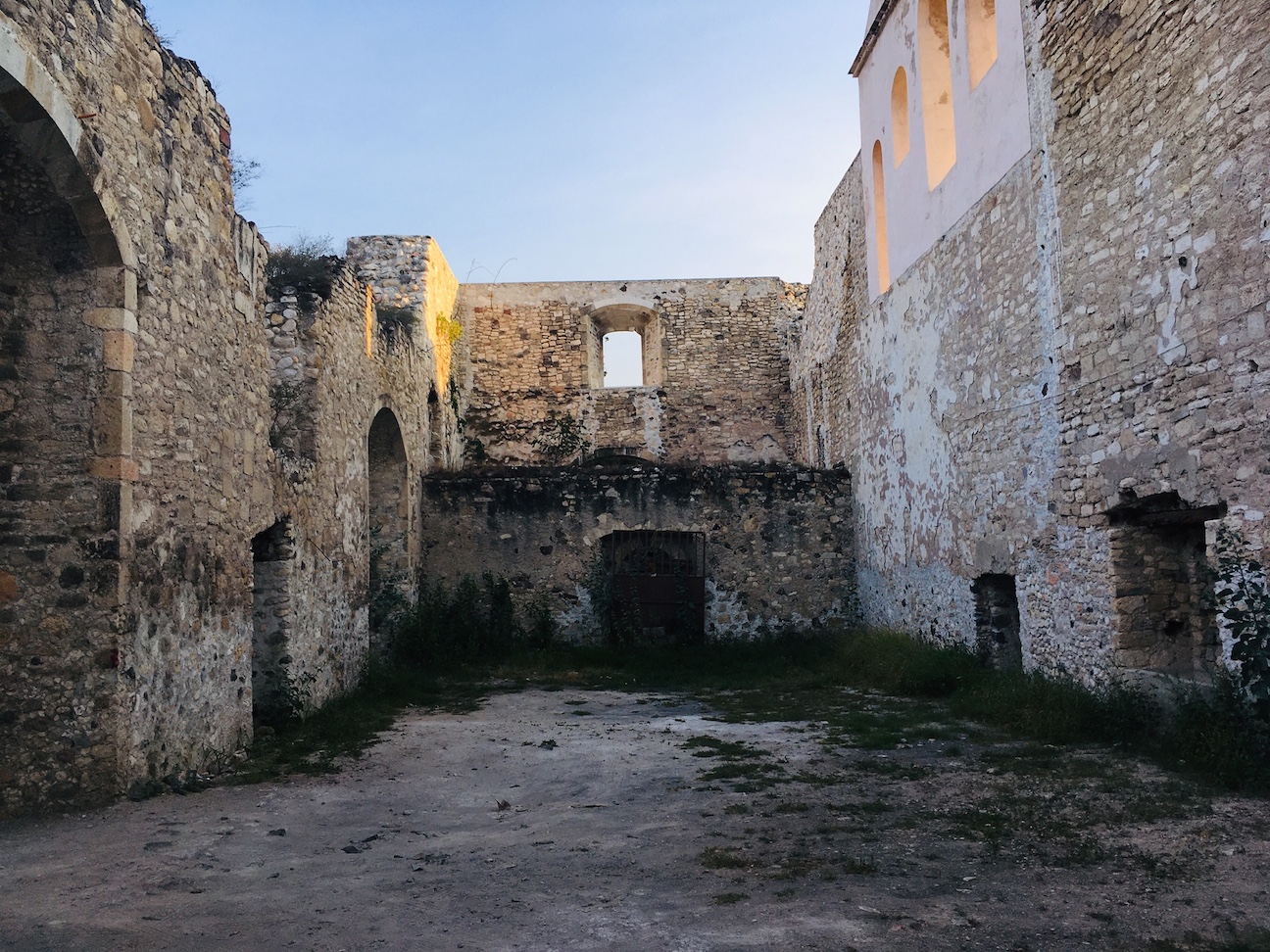The photograph depicts an abandoned and desolate courtyard within the ruins of a stone building, resembling a castle or perhaps a historical European, possibly Italian, structure. The area is barren, with no roof and patches of moss and ivy creeping up the deteriorating walls, some of which are crumbling at the top. Tall, massive stone walls made of stone bricks frame the scene, with archways on the left side suggesting a one-story section, while the right side shows remnants of what was once a two-story area, with windows at different levels indicating former floors. At the center, double wooden doors lie beneath a high window that would have been on the second or third story. The ground is mostly solid dirt, indicating a lack of maintenance, and bares spots with sparse vegetation struggling to survive. Metal bars block what appears to be an entryway, suggesting efforts to preserve some part of the structure. The scene is set under a clear blue sky, adding a stark contrast to the abandoned and silent ruins beneath it.